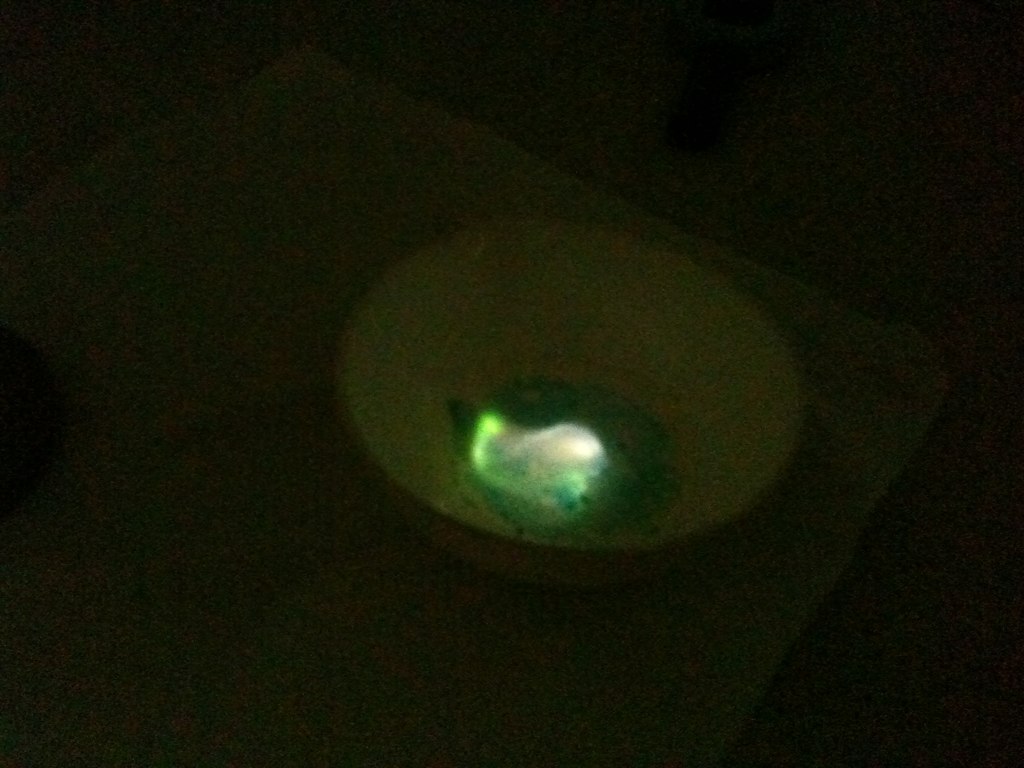The photograph features a dimly lit, out-of-focus scene centered on a highly reflective green rock that appears to be glowing in the dark. The rock, placed on a white porcelain plate with an orange rim, emits a greenish light, which intensifies towards its center, creating a glow-in-the-dark effect. The plate rests on a white fabric table mat, set against a flat, black surface—likely a table—rendered dark due to poor lighting. The background is pitch-black, offering no discernible details or context. The green object's shiny, luminous quality and the overall darkness hint at a mysterious, almost ethereal atmosphere.